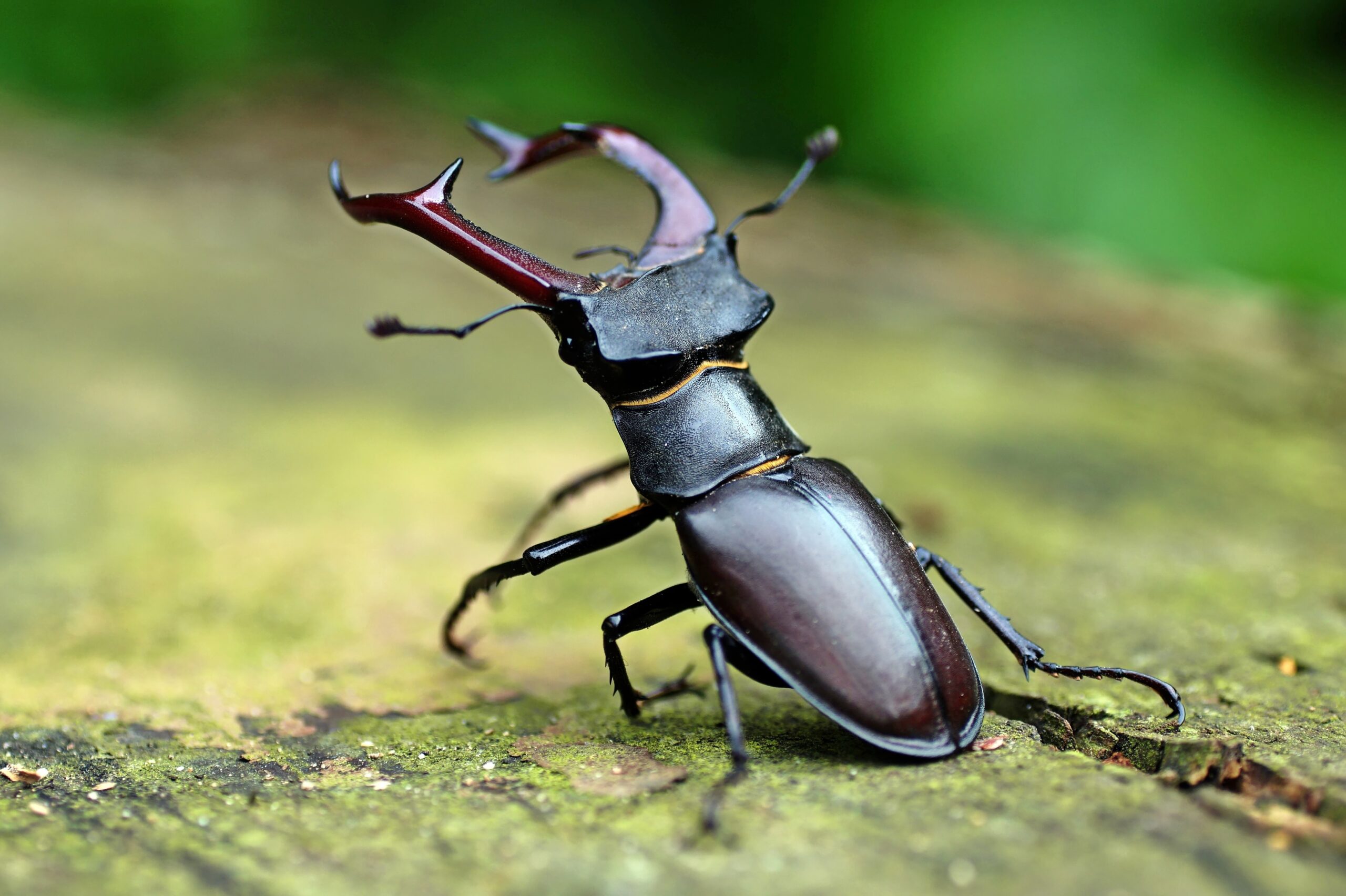This professionally taken macro photograph captures a staghorn beetle in stunning detail. The beetle is predominantly dark reddish-brown, almost black, with a sheen to its carapace. The most striking feature is its large, antler-like mandibles, which are deep burgundy with three sharp points akin to a deer's antlers. Its flat head is adorned with two antennae positioned just above the pincers, and its eyes are visible on either side. A distinctive bright yellow line marks the transition from its head to its thick, black neck, and another yellow marking is present where the neck meets the body. The beetle's abdomen is curved and rounded, coated with shiny brown wings under the carapace. It possesses six spiny legs, though only five are visible in the image.

The beetle is positioned on a piece of wood covered with patches of moss, near a noticeable crack that reveals the texture of the wood. The background is a soft blur of green, likely representing a natural forest setting, providing a contrasting backdrop that accentuates the beetle's form. The detailed shot captures the beetle in what appears to be an alert or defensive stance, adding a sense of dynamism to the image.